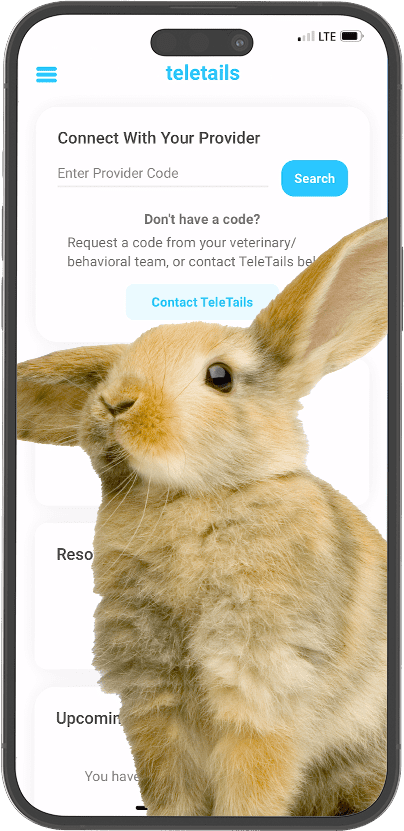The image displays a smartphone screen showcasing a veterinary care application called "Teletails." At the top of the screen, you can see the battery icon and connectivity status in the top-right corner. On the top-left, there is a blue hamburger menu icon. Centered at the top is the name of the business, "Teletails," spelled T-E-L-E-T-A-I-L-S. Below the title, the screen prompts users to "Connect with your provider." 

There is a text box for entering a provider code, accompanied by a blue "Search" button to the right. Underneath the provider code input, a prompt questions, "Don't have a code?" and suggests, "Request a code from your veterinary behavioral team or contact Teletails." The phrase "contact Teletails" is written in blue and appears to be a clickable option.

Taking up the lower portion of the screen is an adorable brown bunny with one ear up and the other to the side, revealing a single brown eye. The bunny is depicted in such a way that partial text appears behind it, with "R-E-S-O" near its chest and "upcoming" near its legs. The bunny's presence adds a charming touch to the screen, making the details about the app somewhat obscured but visually engaging.